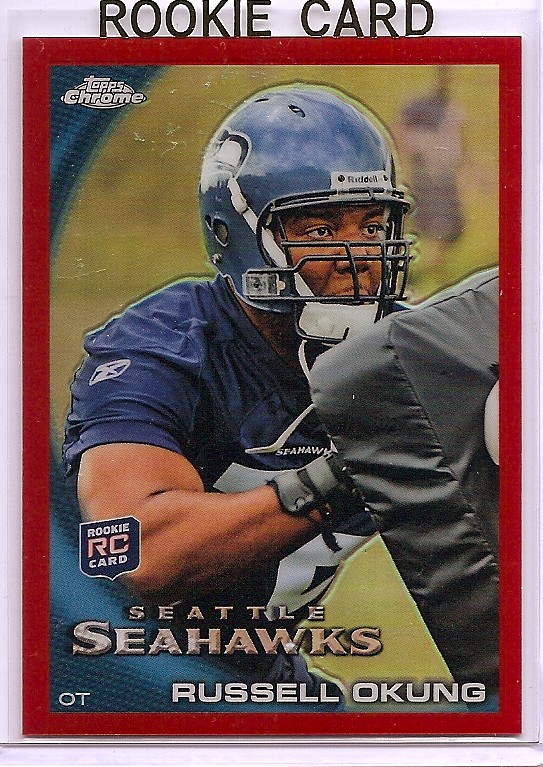The image is a detailed portrayal of a sports trading card, specifically a rookie card, featuring Russell Okung. In the center, a black male athlete, wearing a blue short-sleeved jersey and a matching blue football helmet, is captured either staring to the right or facing forward. He's pushing his arms against a black tackle board. The background of the card is a consistent blue, adorned with white text for clarity, except for the "RC" which stands out in light orange. The top of the card reads, "Topps Chrome" alongside the header, "Rookie Card." Additionally, there is an emblem to the left depicting a seal with the text "Rookie RC Card." The bottom of the card prominently displays the words "Seattle Seahawks" along with "OT Russell Okung." Completing the design, a red border frames the entirety of the card, adding a striking contrast to the image.